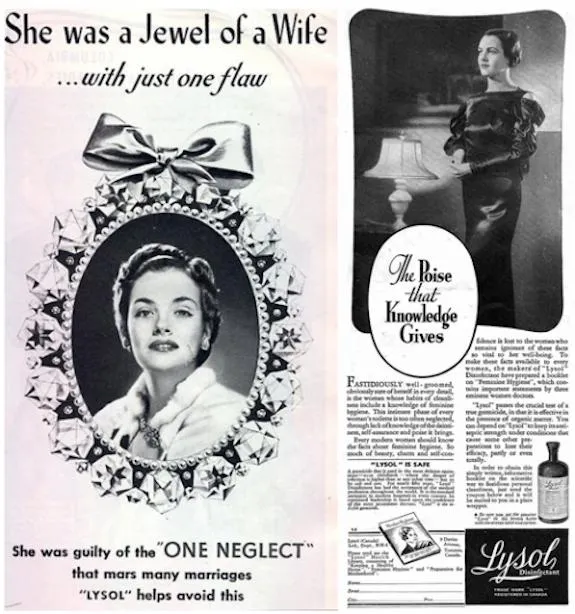This vintage 1930s or 1940s black-and-white magazine advertisement for Lysol features a dramatic layout reminiscent of a true detective story. On the left side, there's a cameo portrait of a white woman with short hair, wearing an ermine mink cape, adorned with a bejeweled bow at the top of the frame. Above the image, the text reads, "She was a jewel of a wife with just one flaw." Below the picture, another line states, "She was guilty of the one neglect that mars many marriages. Lysol helps avoid this."

On the right side of the advertisement, the same woman appears again, this time standing in a stylish black satiny dress beside a vintage lit lamp in a home setting. Encapsulated in an oval speech bubble, the caption reads, "The poise that knowledge gives." Below her, there are approximately five paragraphs of text extolling the virtues and safety of Lysol, encouraging readers to send off for a small booklet. At the bottom left, there is a mail order form to request this informational booklet, further indicating the ad's focus on marital harmony and domestic sanitation.